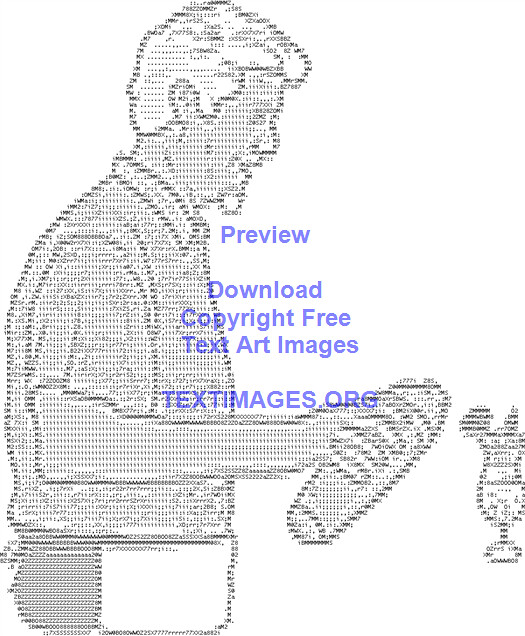This digital artwork showcases a tall rectangular ASCII art image drawn using various key symbols such as dots, dashes, commas, and semicolons, all in tiny black font. The piece features a man with white hair, a white goatee, and a stylish haircut, visible from the waist up and facing right. He is dressed in a gray collared short-sleeved t-shirt and a white apron, holding a drink shaker as he prepares to pour a cocktail into a glass. The cocktail glass, positioned at the bottom right of the image, features a stem and base, adorned with an umbrella and a piece of fruit. The entire image is set against a white background, and the text "Preview Download Copyright Free Text Art Images" along with "textimages.org" appears in light blue and purple fonts.